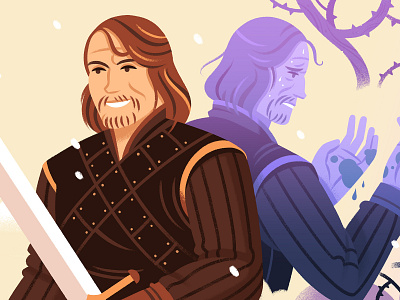This cartoon image depicts a Caucasian man with long brown hair, a beard, and a mustache, dressed in early 1800s, late 1700s attire. He is wearing a brown jacket with striped sleeves and a crisscrossing lapel or holster strap across his chest. He stands smiling, facing forward, holding a white sword in his left hand. Behind him is a mirrored, shadow-like image of himself in shades of purple and blue, looking down at his hands which appear to be covered in blood. The reflected figure has an expression of chagrin. The background is cream-colored, with what seems to be a thorny purple tree branch positioned above the man's head on the right.